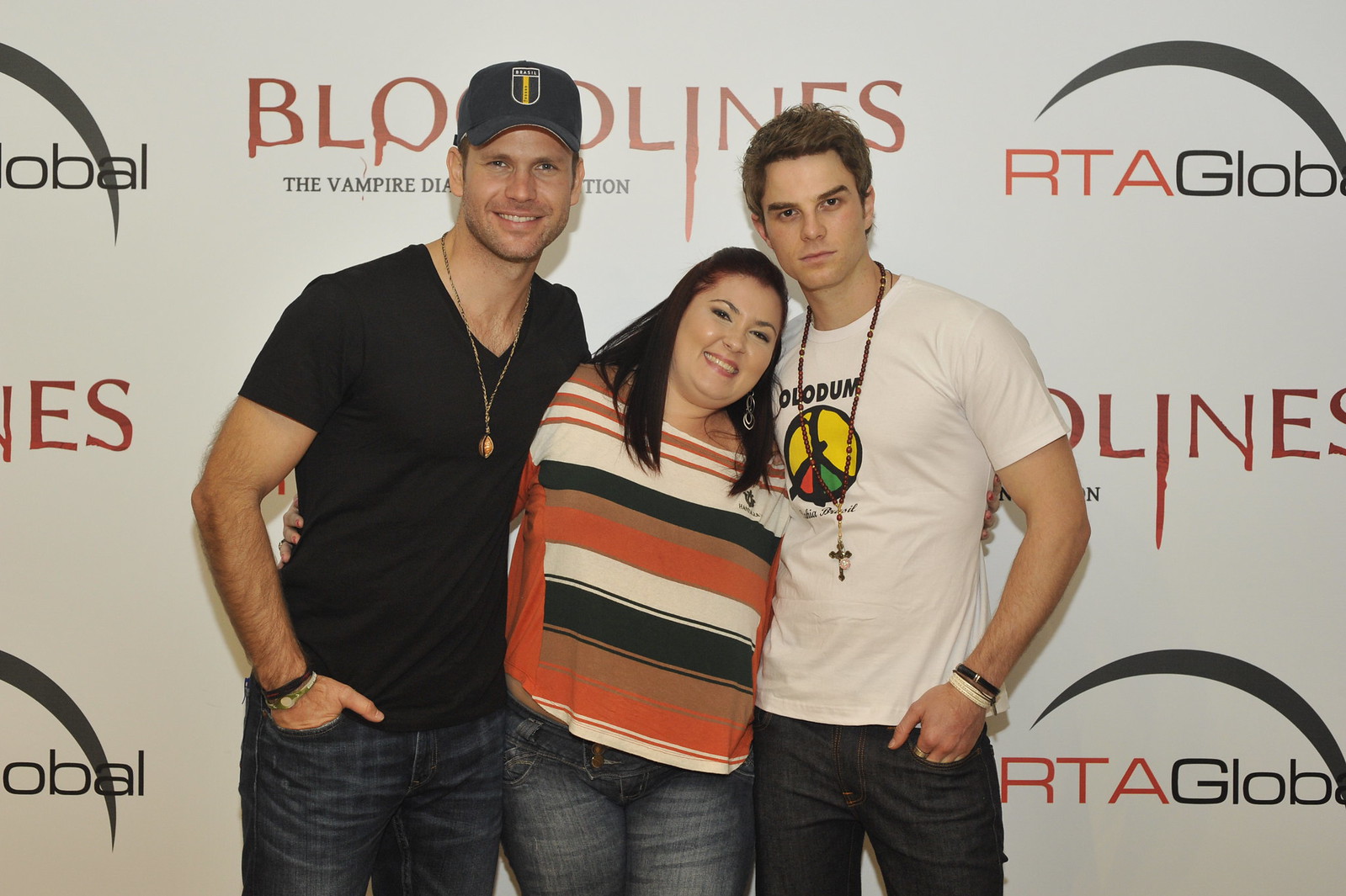This photograph captures three individuals closely posing for a picture against a backdrop decorated with text and icons related to "Bloodlines," "RTA Global," and "The Vampire Diaries edition." The man on the left is notable for his black hat, black t-shirt, bracelets, and blue jeans; a necklace glints around his neck. He stands with one hand in his pocket, sharing a smile. In the center is a woman with long brown hair, who leans her head against the man on the right. She is dressed in a colorful striped t-shirt with shades of orange, white, black, and brown, paired with blue jeans; her smile and relaxed posture suggest a sense of camaraderie. The man on the right, also smiling, sports a white t-shirt displaying a peace symbol in yellow, red, and green, as well as text that partially reads "O-D-O-D-U-M." He is adorned with rosary beads and bracelets, and wears black pants. Both men and the woman are united by their friendly embraces and forward-facing stance, positioned centrally in the image. This indoor setting, reminiscent of a fan meetup or red carpet event, is illuminated by the vibrant colors and iconic references on the backdrop, enhancing the celebratory mood of the photo.